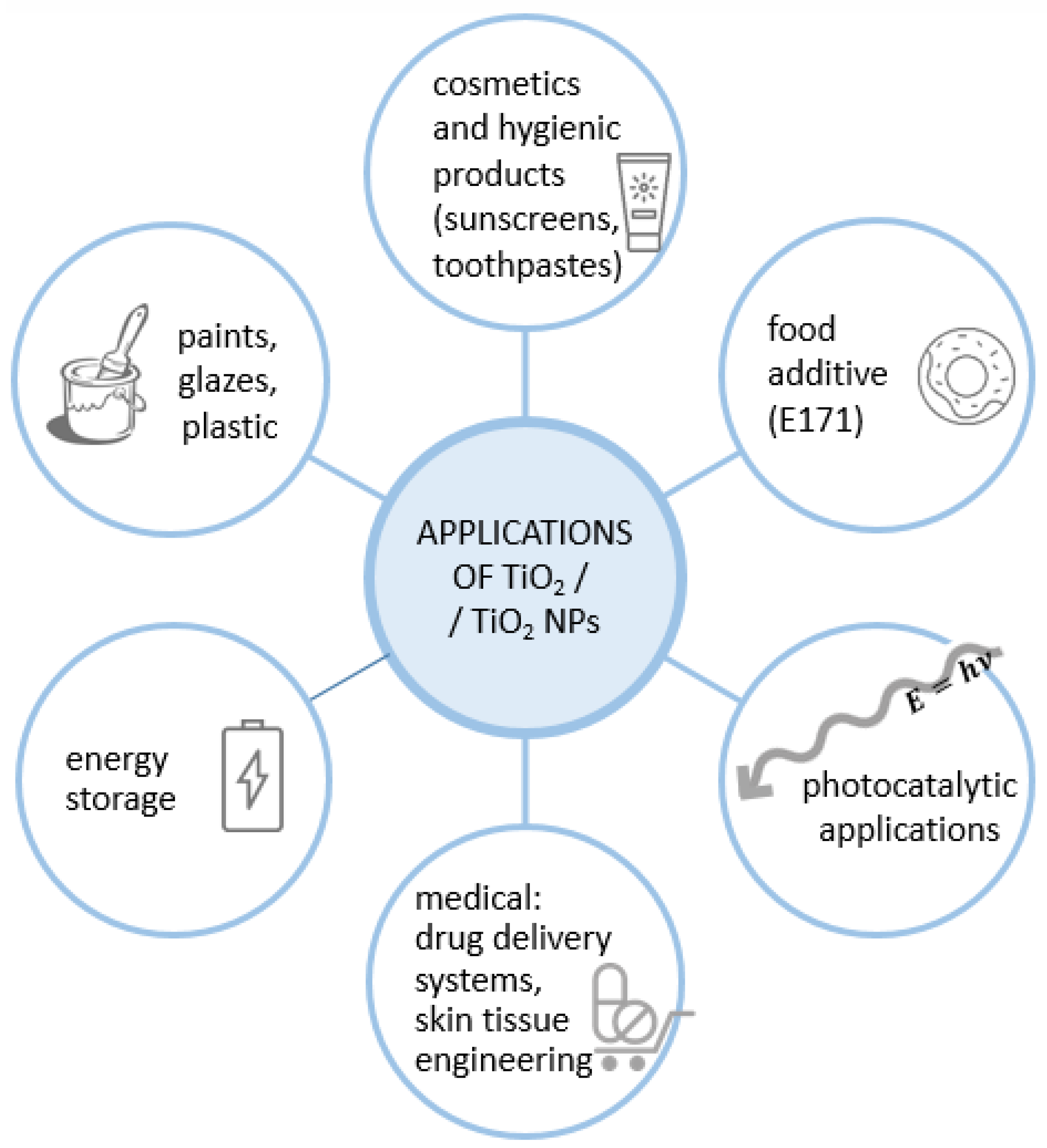This vertical image is a detailed diagram with a white background and no border, presenting the "Applications of TiO2/TiO2 NPs" in the central blue-outlined circle. Surrounding this central circle are six smaller circles, each linked by blue lines, displaying text in black. The surrounding circles, each with a white background and a blue border, illustrate various applications of TiO2. Starting from the top, one circle lists "Cosmetics and Hygienic Products," including an icon of a sunscreen package and mentions "Sunscreens" and "Toothpaste." Moving clockwise, another circle is labeled "Energy Storage." The next circle details "Medical Devices" and "Drug Delivery Systems." Further along, another circle indicates "Skin Tissue Engineering" and "Photocatalytic Applications." Another reads "Food Additives," specifically "E171." Finally, the last circle notes "Paints, Glazes, and Plastics" with an illustration of a bucket and paintbrush. The colors used within the image include light blue, darker blue, white, black, and gray.